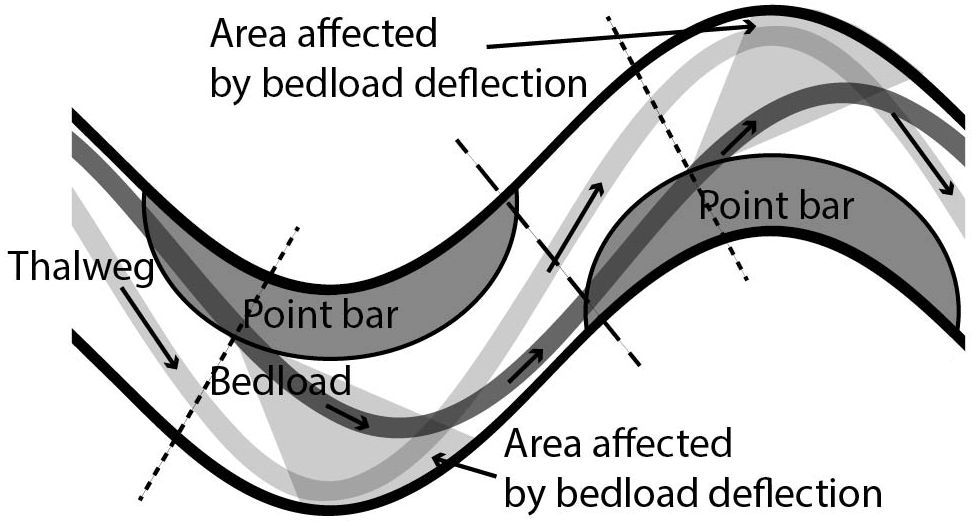This monochrome graphic diagram, possibly related to engineering or geology, illustrates a detailed representation of wave-like motion. The black and gray wave, divided into sections by dashed lines, features numerous labeled areas. Key designations include "VAL," "WEG," "point bar," and "bed load," with areas repeatedly marked as "affected by bed load deflection." Distinct crescent moon shapes along the curvatures are labeled as "point bar." Arrows throughout the diagram indicate directionality. The composition is intricately segmented with specific positioning of the terms, clearly demarcating different phenomena within the wave structure.